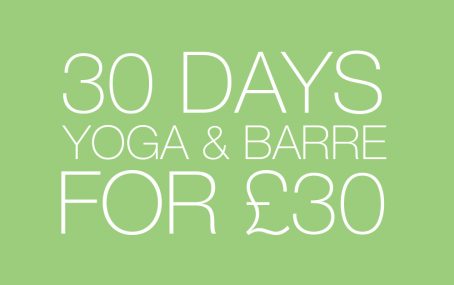A minimalistic banner ad for a yoga studio displayed against a soothing sage green background. The ad features clean, thin, white sans serif text, centrally justified, that reads: "30 days yoga & barre for £30." Notably, the word "and" is replaced with an elegant ampersand. The phrase "yoga & barre" is rendered in a slightly smaller font size than the remaining text, subtly emphasizing the offer. While the ad provides no specific details such as the studio's name, address, or contact information, it suggests this banner is likely designed for placement within the company's own website, where further information is available. This ad, simple yet effective, clearly communicates a promotional offer tailored for audiences in England.